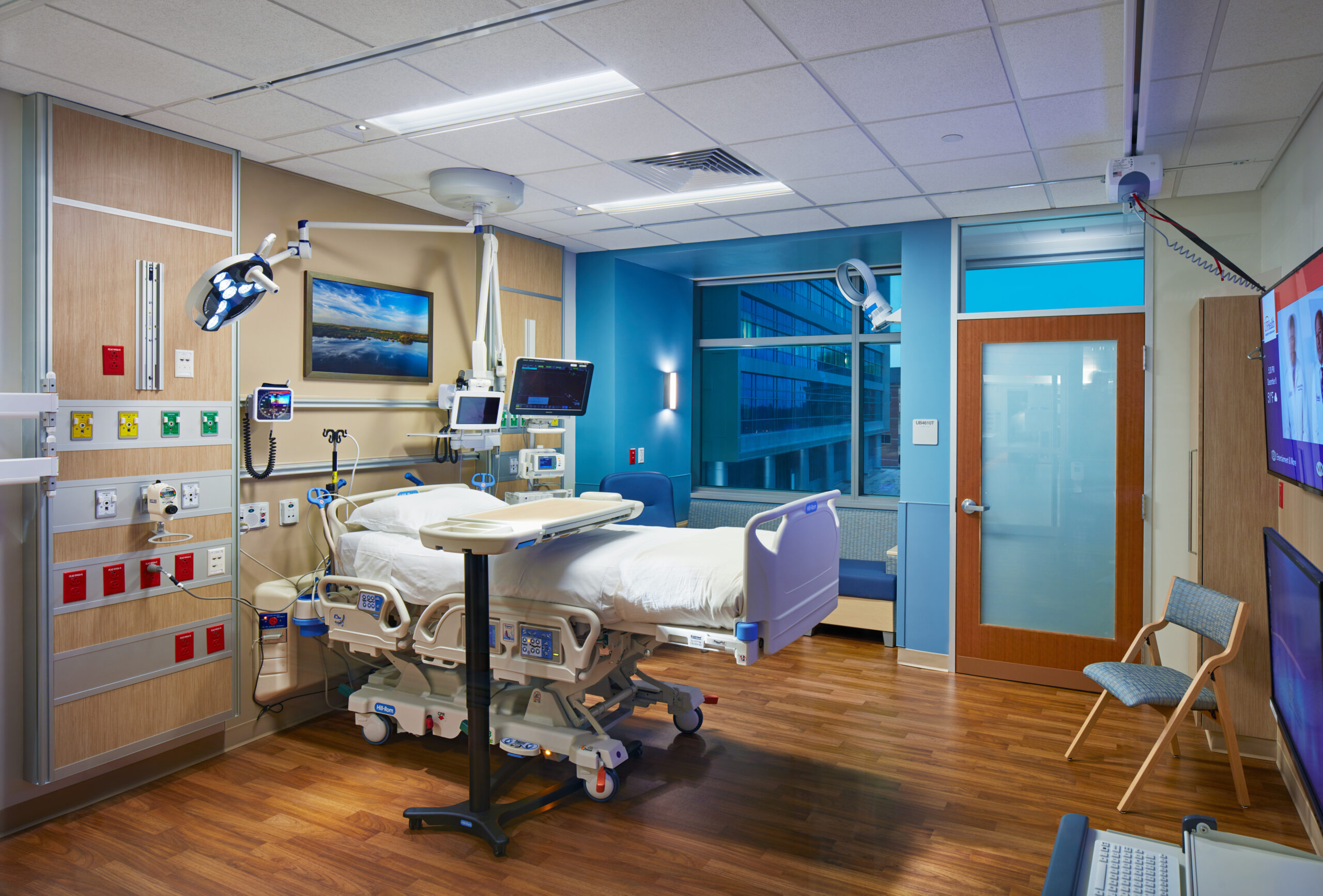The photograph captures a well-lit, empty hospital room with a distinct medical ambiance. The room features a brown hardwood floor and a hospital bed positioned in the middle-left of the image, elevated and equipped with wheels for mobility. Above the bed, there's a serene painting depicting blue sky and water. Notably, the room is outfitted with various medical equipment, including numerous monitors and screens situated near the bed, along with an array of plugs and outlets on the wall behind it for essential medical devices. 

To the right of the bed, there's a special blue light machine, adding to the room's high-tech medical environment. Across from the bed, a television hangs on the wall, with what appears to be a secondary screen or monitor positioned below it. 

The room also includes practical furnishings such as a hospital tray and a computer station located in the lower right corner. The space is complemented by a blue chair with wooden legs, offering a place to sit. Additionally, a glass door and a window provide views of another part of the hospital building outside, characterized by large glass windows. The overall design exudes a warm yet highly functional atmosphere, ready to accommodate patient care.